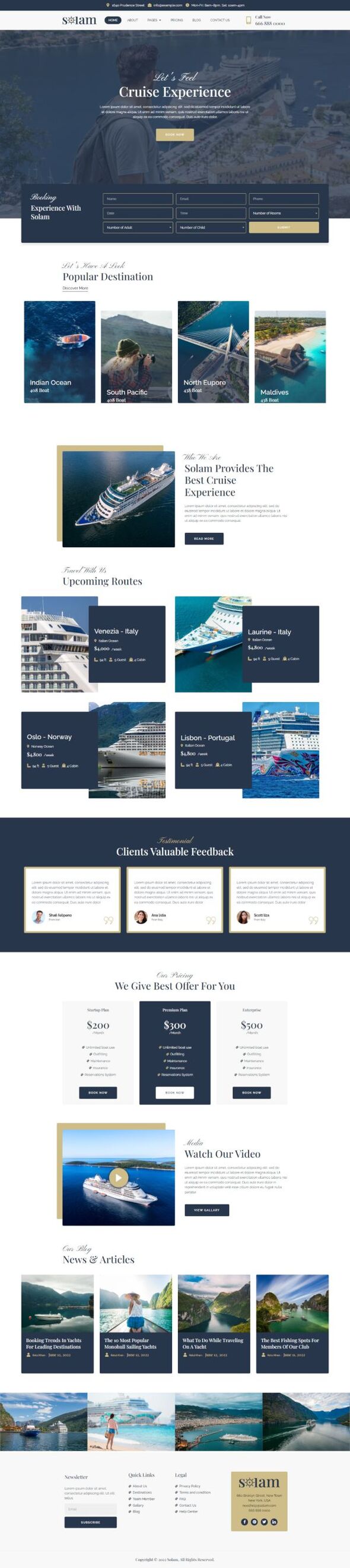**Experience the Ultimate Cruise Adventure with SLAM Cruises**

The SLAM cruise brochure invites you to immerse yourself in a world of luxurious maritime travel with Solom. The brochure cover showcases a bustling dock filled with cruise ships arriving and departing, symbolizing the beginning of countless unforgettable journeys.

**Popular Destinations:**
SLAM Cruises offers an array of popular destinations including the stunning Indian Ocean, the serene South Pacific, the picturesque North European region, and the idyllic Maldives. Picture yourself on the pristine, sandy beaches of the Maldives, with turquoise waters stretching endlessly around you—truly a paradise on earth.

**The Solom Cruise Experience:**
A striking image of a Solom cruise ship highlights the exceptional cruise experience provided by Solom. The ship's innovative design promises comfort and luxury, ensuring your voyage is as enjoyable as the destinations themselves.

**Upcoming Routes:**
- **Venezuela to Italy**
- **Lorraine to Italy**
- **Oslo, Norway to Lisbon, Portugal**

The cruise ships boast vibrant and artistic hulls adorned with murals of waves, suns, and bright colors such as hot pinks, greens, and yellows, making each ship unique and visually captivating.

**Exclusive Offers:**
The brochure also highlights client testimonials and valuable feedback. SLAM Cruises offers exclusive rebates based on your stateroom choice:
- $200 rebate for standard staterooms
- $300 rebate for deluxe staterooms
- $500 rebate for premium suites

**Visual Highlights:**
A video link provides a visual tour of the cruise ships sailing through majestic blue waters, inviting you further into the SLAM cruise experience.

**Additional Yacht Services:**
Beyond cruising, SLAM offers yacht services, featuring tips on activities while sailing, the best fishing spots for club members, and insights into the latest yacht design trends. While the brochure includes fewer images of yachts compared to cruise ships, the information remains compelling.

The brochure concludes with an elegant image of a lady standing on a sunlit beach, with a majestic cruise ship anchored nearby, encapsulating the essence of a dream vacation.

Explore new horizons and discover unparalleled luxury with SLAM Cruises. Your perfect maritime adventure awaits.